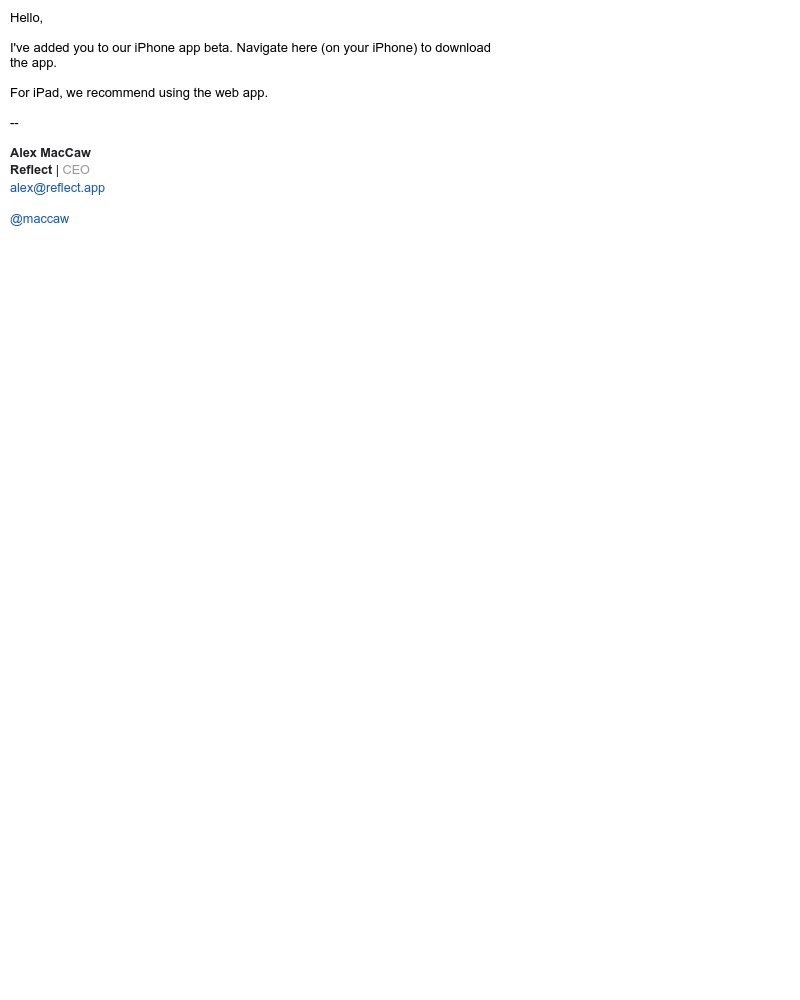The image depicts a clean, minimalist design aimed at guiding users on how to access the beta version of an iPhone app. The background is entirely white, emphasizing simplicity and readability. Text instructions are prominently displayed in black, leading users through the process of downloading the app. Key URLs such as "alex.reflect.app" and "appmccaw" are highlighted in blue to draw attention. For iPhone users, a specific navigation path is suggested to download the app. For iPad users, visiting the webpage at "alex.reflect.app" or "appmccaw" is recommended. The repetition of certain text elements and the color-coded URLs ensure clarity and ease of access for the user.